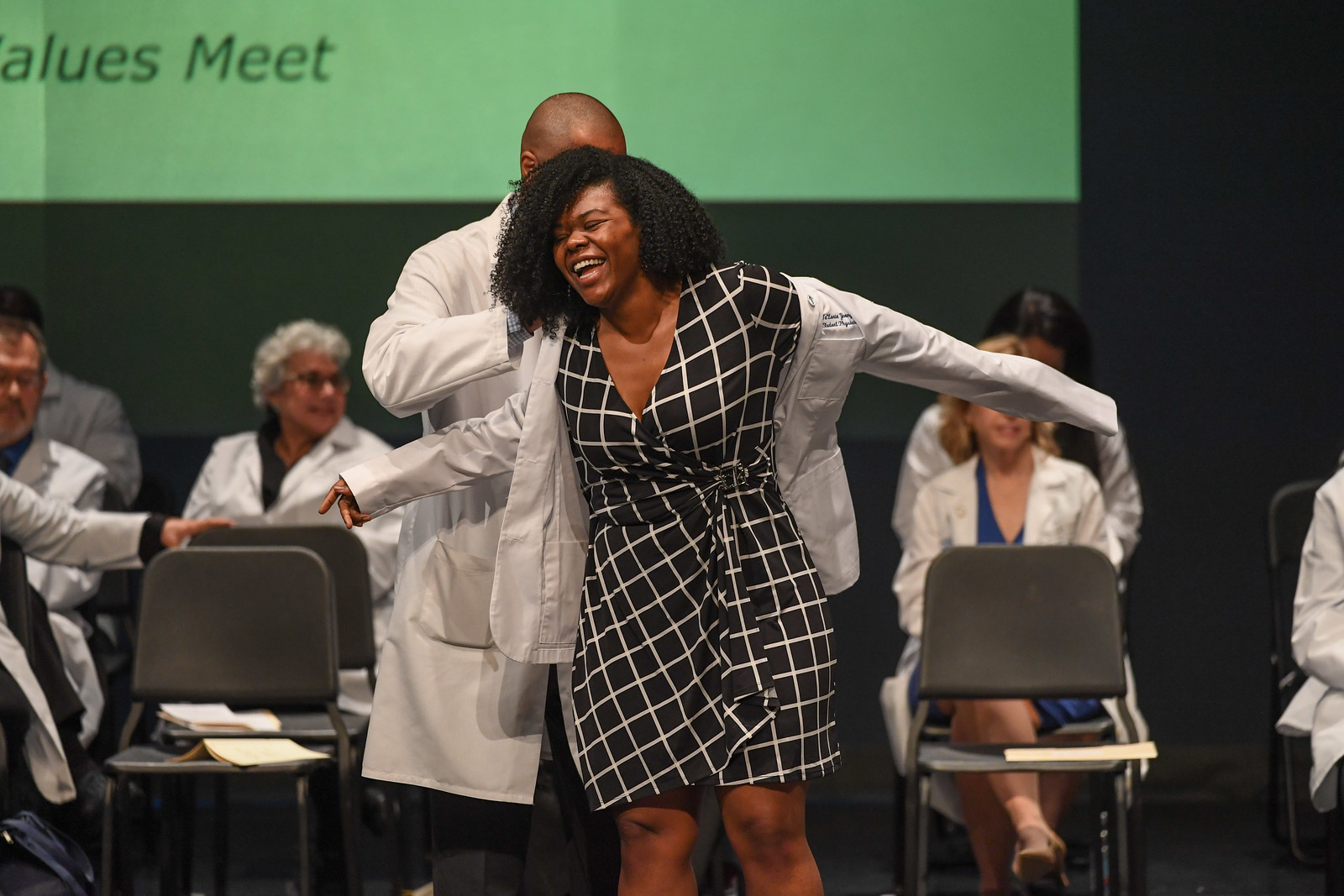In this photograph, a pivotal moment is captured as a woman stands on stage, receiving her white coat in what appears to be a white coat ceremony, a significant event in the medical community. She has short, very curly black hair and is dressed elegantly in a black dress with white lines. A bald man, who appears to be African American, is assisting her in putting on the white coat, signifying her entry into the medical profession. Seated behind them are several individuals, also wearing white coats, suggesting they are either established doctors or medical professionals witnessing the ceremony. The atmosphere exudes a sense of accomplishment and anticipation, highlighting the importance of this milestone in the woman's journey to becoming a doctor.